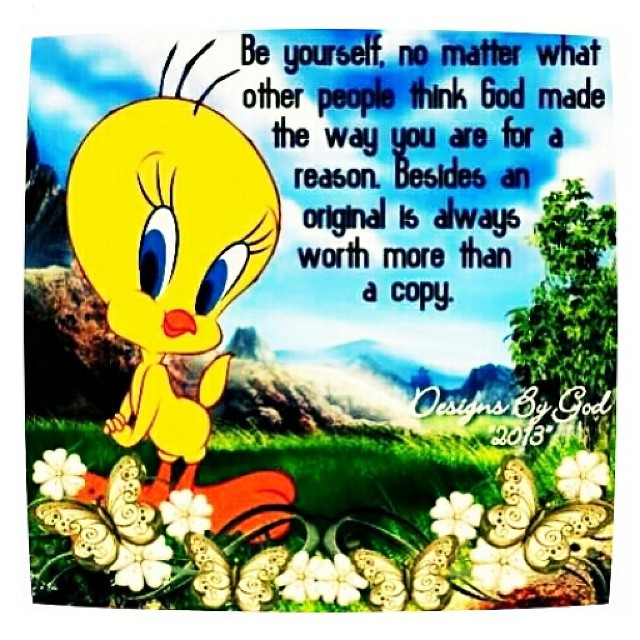The image is a vibrant and detailed illustration that appears to be either a scanned handout or a postcard, designed as a motivational message meant to be shared online. The primary scene is a colorful outdoor landscape featuring a grassy field densely populated with various shades of green, adorned with white and goldish-yellow flowers, and butterflies that display intricate patterns of black and dark brown lines and dots.

In the foreground on the left side, there is the iconic cartoon character Tweety Bird. Tweety Bird is depicted with its classic big blue eyes, yellow feathers, and reddish-orange beak and feet, standing with its little cartoon hands folded in front. Behind Tweety Bird, a picturesque landscape unfolds, including a lake, mountains, and trees set against a blue sky with scattered white clouds. To the right side of the image, distant misty mountains add depth to the scene.

At the top right corner, inspirational text in black reads: "Be yourself no matter what other people think. God made you the way you are for a reason. Besides, an original is always worth more than a copy." Below this text, in a white scripted font, it states: "Designs by God 2013," which appears possibly with an asterisk or quotation marks partially obscured by the background. Despite the vivid and inspirational design, there is no visible credit to Warner Brothers, who owns the copyright to Tweety Bird. The entire composition exudes a motivational and uplifting message, set against a richly detailed, colorful landscape.